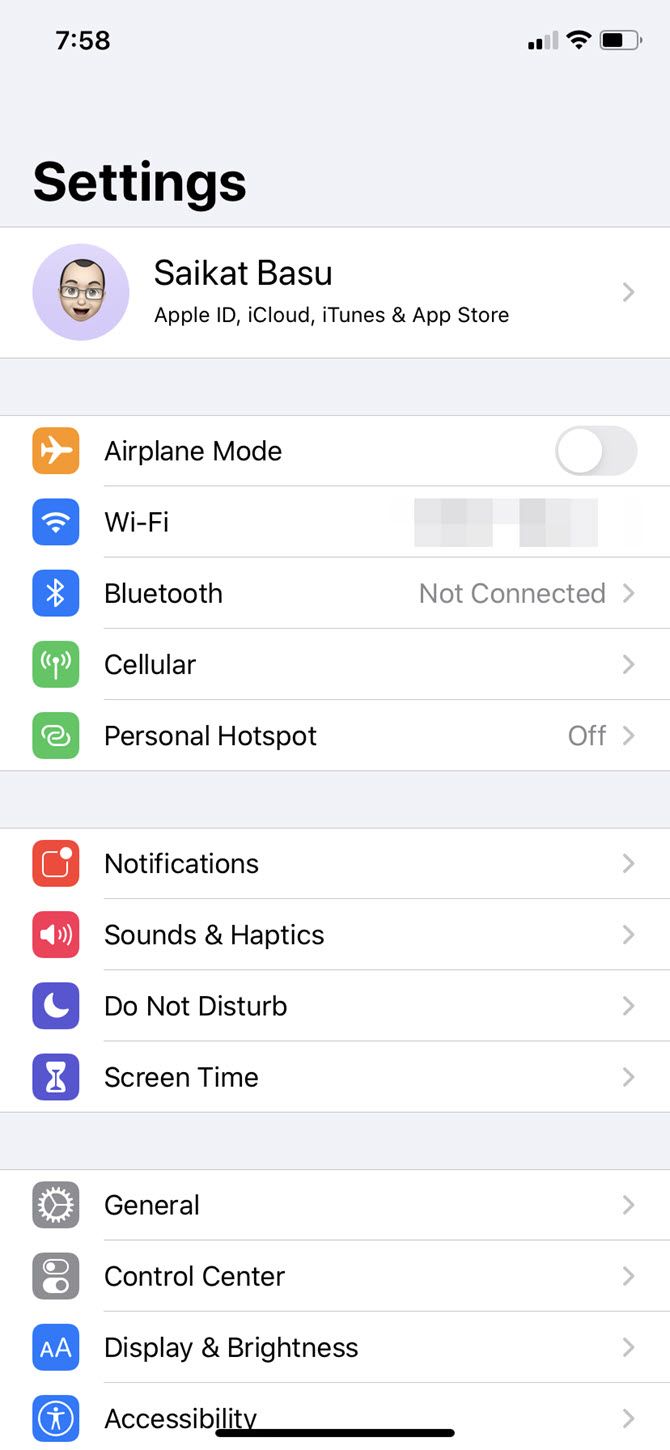A user is navigating their iPhone settings, signed in as "Saikat Basu." The screen displays a typical settings interface on a white background, with each setting accompanied by its respective icon. The user’s avatar is depicted as a Caucasian male with a receding hairline and glasses.

The screen includes options such as Airplane Mode (toggle switch), Wi-Fi (network name blurred), Bluetooth (not connected), Cellular, Personal Hotspot (off), Notifications, Sounds & Haptics, Do Not Disturb, Screen Time, General (gear icon), Control Center, Display & Brightness, and Accessibility (icon resembling the Vitruvian Man). The battery level is a little over half, and the time displayed is 7:58. Airplane Mode, Wi-Fi, and Bluetooth settings are prominently featured at the top of the list, indicating essential connectivity options.